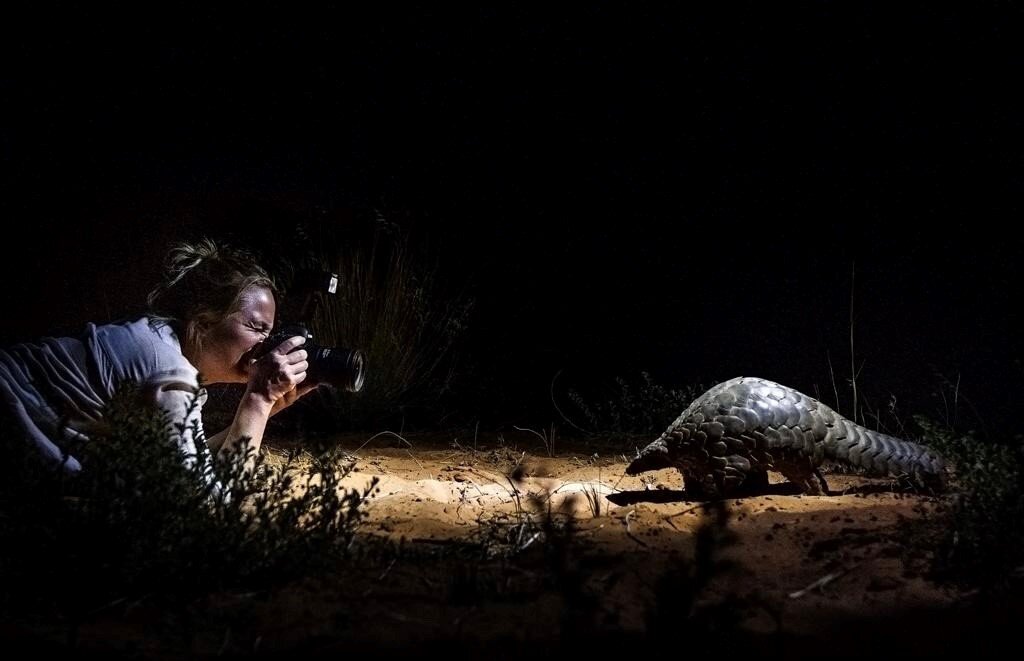In this striking nighttime photograph, a woman with light blonde hair pulled into a ponytail kneels down on her elbows on the left side of the frame, intently focusing her large digital camera on a curious creature before her. Clad in a white long-sleeved shirt rolled up to her elbows and poised against the dark landscape orientation backdrop, she directs her lens toward a pangolin—a mammal often mistaken for an armadillo. The pangolin is bathed in a spotlight that dramatically illuminates its pointy head, large scales, and long, thick tail, emphasizing its unique, armor-like appearance. Both subjects are captured in profile against a pitch-black background, punctuated by a single straggly plant and sparse grass beneath them, their forms accentuated by the light that casts them vividly into relief from the enveloping darkness.